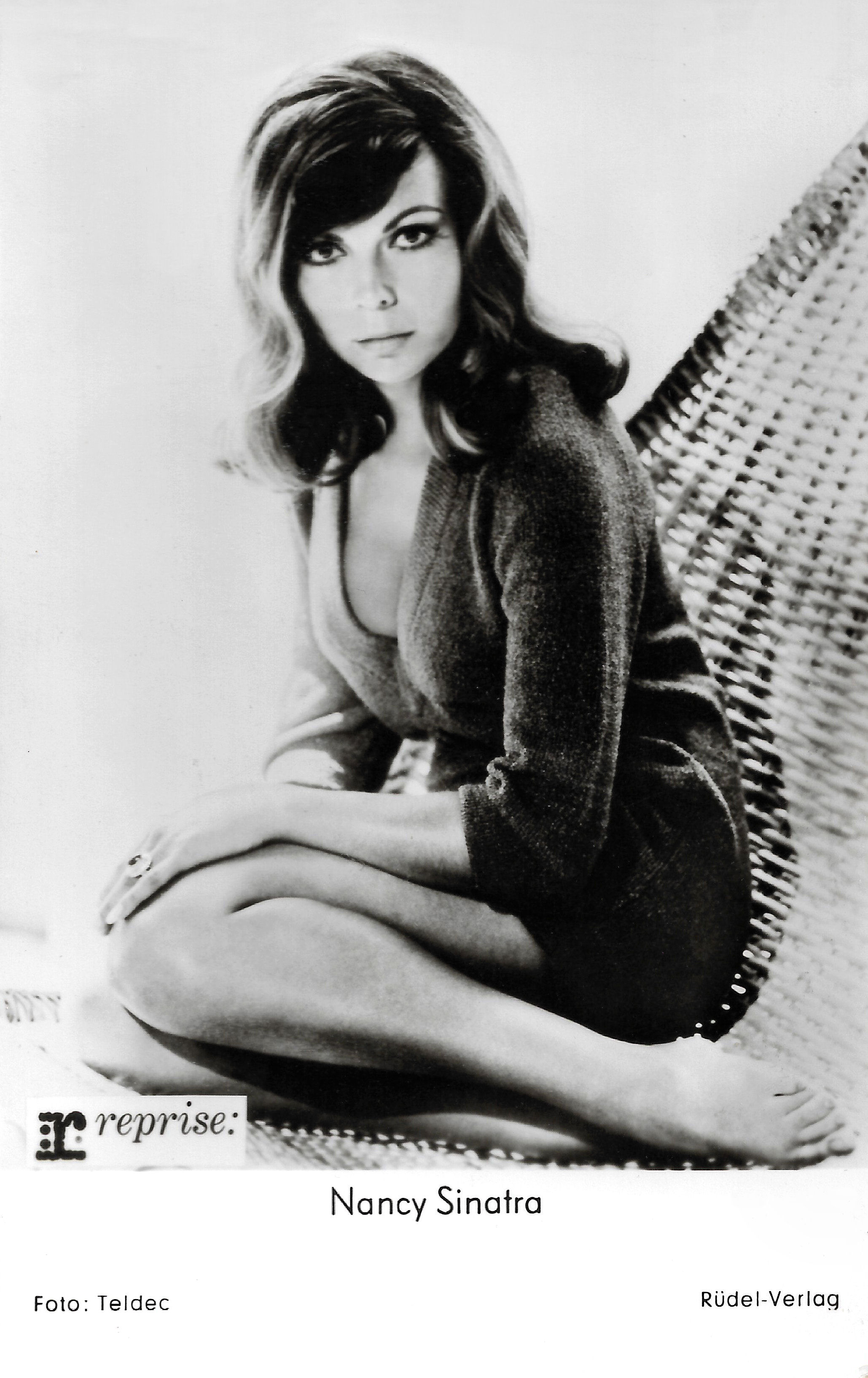This black and white photograph features Nancy Sinatra, as stated in the black text at the bottom of the image. Nancy, the daughter of Frank Sinatra, is seated on what appears to be a hammock with a textured fabric, which, interestingly, rests on the ground. Her legs are bent at the knees, folded underneath her, revealing most of her left leg up to her thigh due to the very short skirt she is wearing. The dress is casual, with some describing it as a black or red terry cloth. She sports long brown hair falling to her shoulders and wears dark, bold eye makeup typical of the 1960s, gazing directly at the camera with her hands posed on her knees. She is barefoot. The background of the photograph is either gray or white, and Nancy is centrally positioned. Additional text beneath her name includes the word "Reprise," likely referencing the record company, and other unreadable text in a different language. There's also a ring visible on her left finger and a possible chair seen behind her. This detailed portrait captures the essence of Nancy Sinatra's style and era.